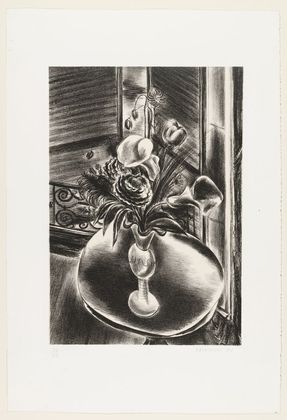This is a black-and-white pencil drawing that features a small round table situated by a window, presumably on the second floor as suggested by the visible metal railing outside. The window behind the table has shutters, adding depth and context to the scene. On the table stands a vase holding a diverse bouquet of flowers, including roses, lilies, and possibly tulips. The illustration employs an abstract style, with smudged shading creating shadows and depth, and while it is not photorealistic, it effectively captures the essence of each element. The composition centers the vase with flowers in the middle, with the table at the bottom and the window at the top, framed by the balcony's railing and the open window behind it.